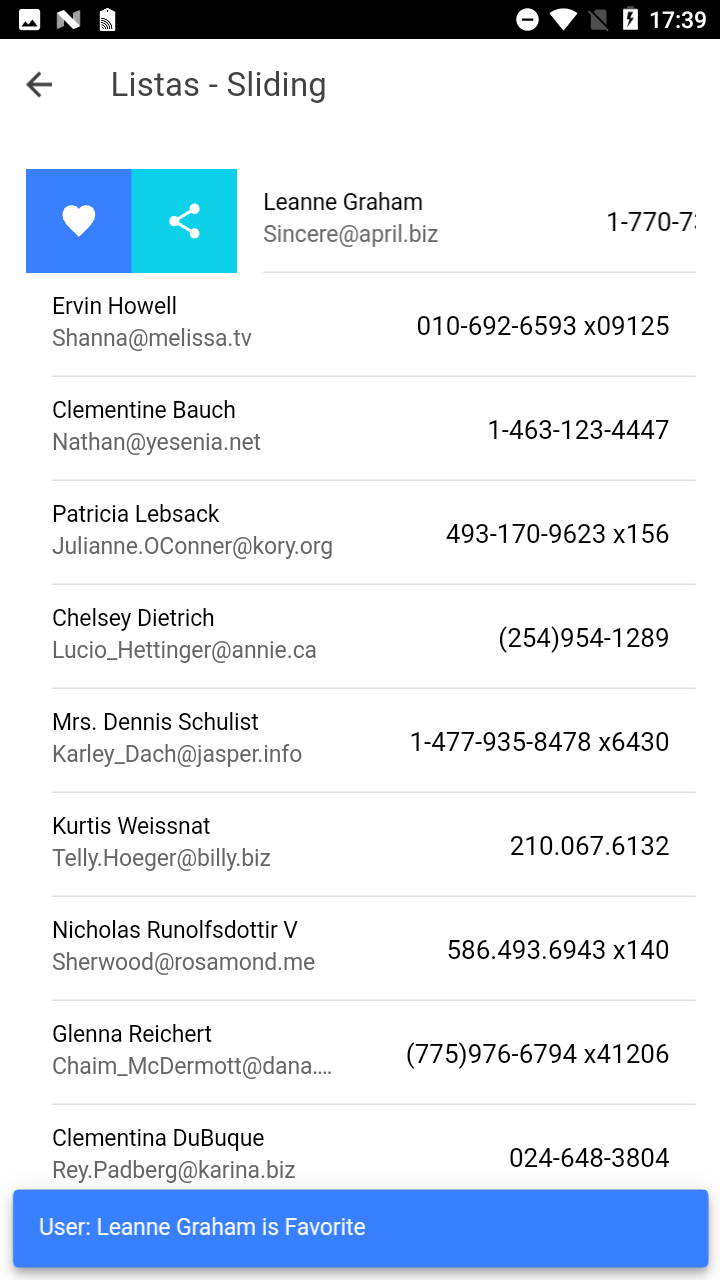A detailed screenshot from a mobile application, likely named "Listus," captured at 17:39. Clearly visible, the mobile interface showcases standard icons: a Wi-Fi symbol, battery indicator, and the time in the top black bar. Just beneath this, within an all-white backdrop, are a back arrow and the title "Listus - sliding." Below this title, two icons—a heart and a share symbol—are present, suggesting options for favoriting and sharing.

The main content area displays a list of contacts, resembling an address book. The first contact, Leanne Graham, shows her email as "sincere@april.biz" and a portion of her phone number, with further digits obscured. The display indicates Leanne Graham's selection, emphasized by a blue highlight and a note at the bottom stating "User Leanne Graham is favorite."

Following Leanne Graham, additional contact names include Irvin Howell, Clementine Balch, Patricia Lebsack, Mrs. Dennis Shulist, and Curtis Weissnacht with listed email addresses and partial or full phone numbers. The structured layout and clean design suggest a user-friendly interface for managing contacts.